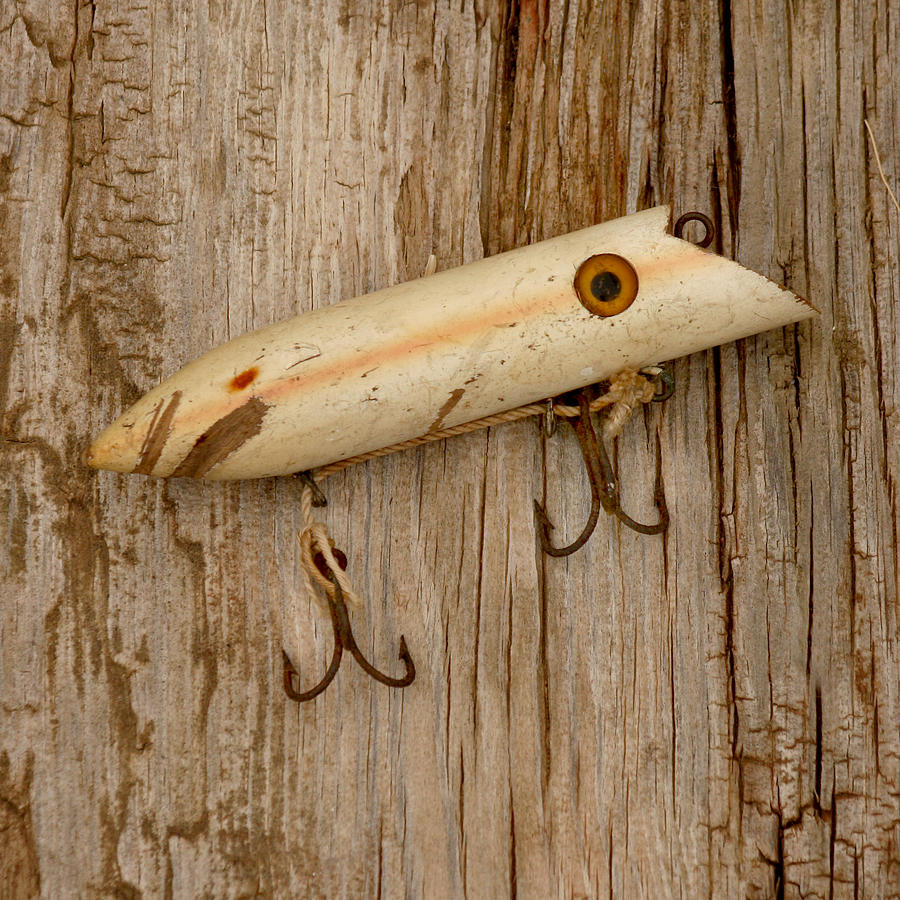The photograph captures a weathered fishing lure positioned centrally on a worn, wooden surface, likely a dock or table. The fishing lure, which appears to be made of wood or a wooden-like material, has clearly aged, displaying a dark ivory hue with a thin orange stripe running down its center. The lure features two rusted fish hooks at its bottom, each with two sharp prongs, and a small circular bracket at the top, possibly for hanging or attaching to a fishing line. The overall color palette includes variations of brown and yellow, amplifying the rustic and vintage feel of the image. Notably, there is no text identifying the object, and no people or animals are present in the scene.